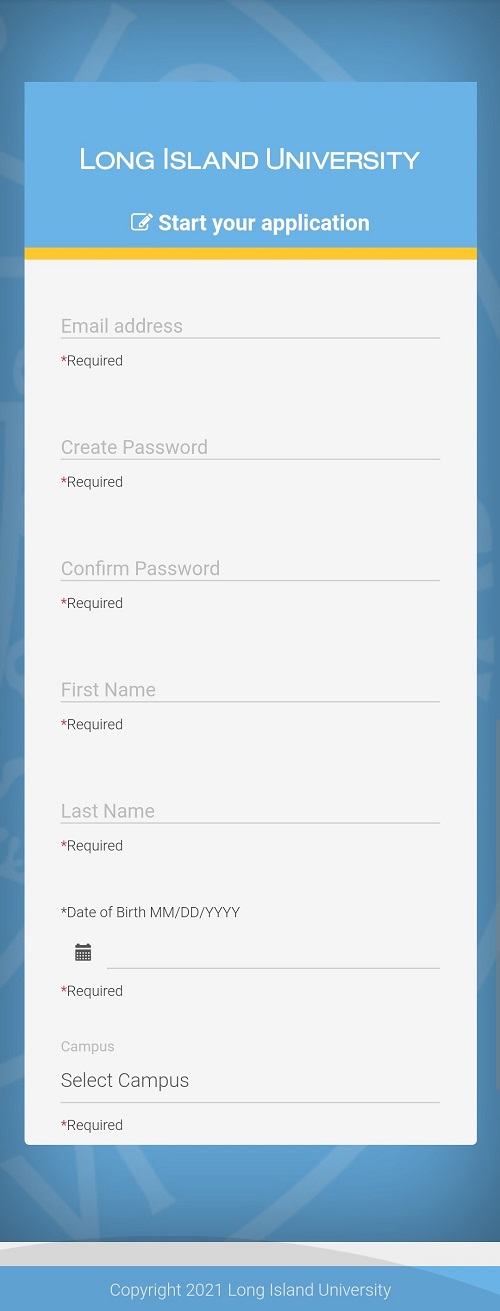The image features an application form for Long Island University set against a predominantly blue background. The central area, where applicants input their information, stands out with a clean white background. At the top of the form, within a light blue square, "Long Island University" is prominently displayed in white text. Directly below this, there is a small icon of a pencil inside a square with the text "Start Your Application" next to it.

The form includes several fields, each labeled as required with an asterisk (*): 
- "Email Address"
- "Create Password"
- "Confirm Password"
- "First Name"
- "Last Name"

Additionally, there is a section for entering the "Date of Birth" which includes dropdown menus for the month, day, and year, complemented by a clickable calendar icon to facilitate date selection. The form also requires applicants to "Select Your Campus."

At the very bottom of the image, within a small blue square, the text "Copyright 2021 Long Island University" is displayed.